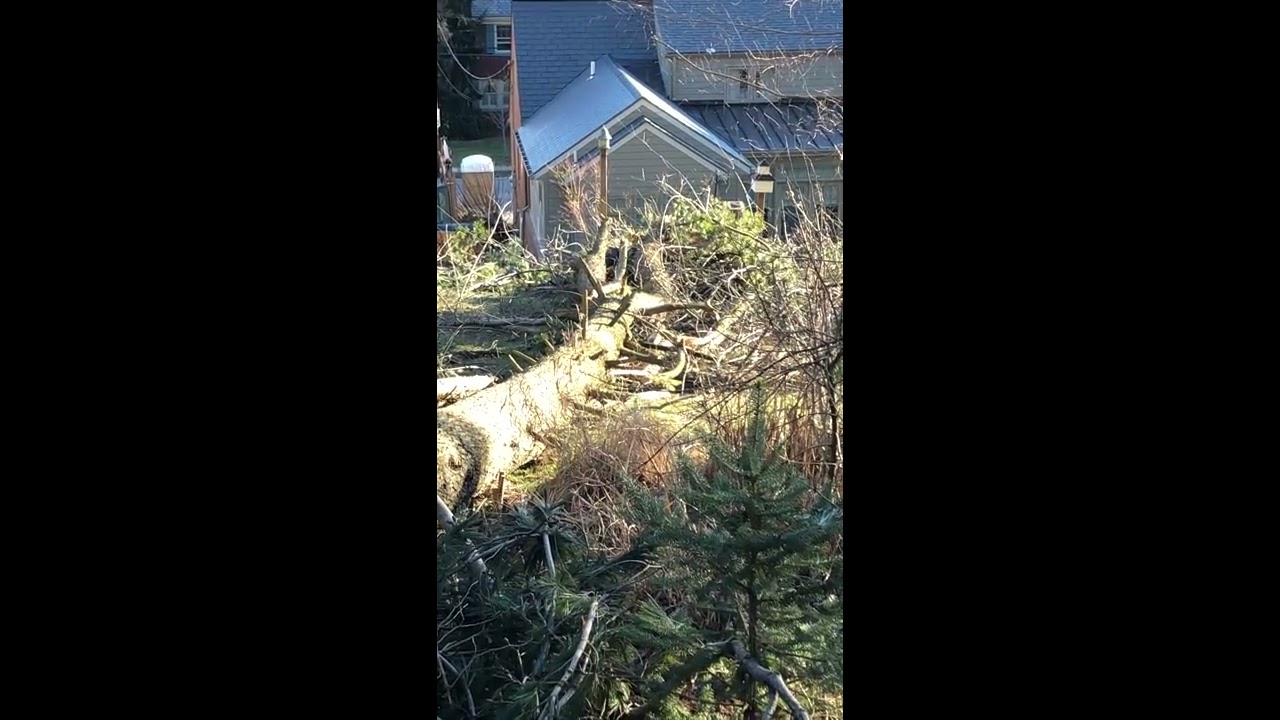The photograph captures an outdoor setting bathed in daytime sunlight, featuring a felled tree lying amidst wild, unmanicured green foliage that surrounds a dirt-covered walkway. The felled tree, likely downed by a storm, dominates the scene with its branches cut off and scattered around. In the background, a gray gabled house with a pole next to it stands prominently, flanked by a fence. Behind this house is a single-story building with a flat roof. The image has a vertical orientation, forming the center panel of a triptych, with black panels on both sides. An electrical wire extends across the scene's upper left, and the surrounding area, characterized by flattened and broken brush, suggests a recent upheaval. The photo appears to be taken from an elevated position, leading downhill towards the house, capturing the atmosphere of a quiet residential area post-storm.